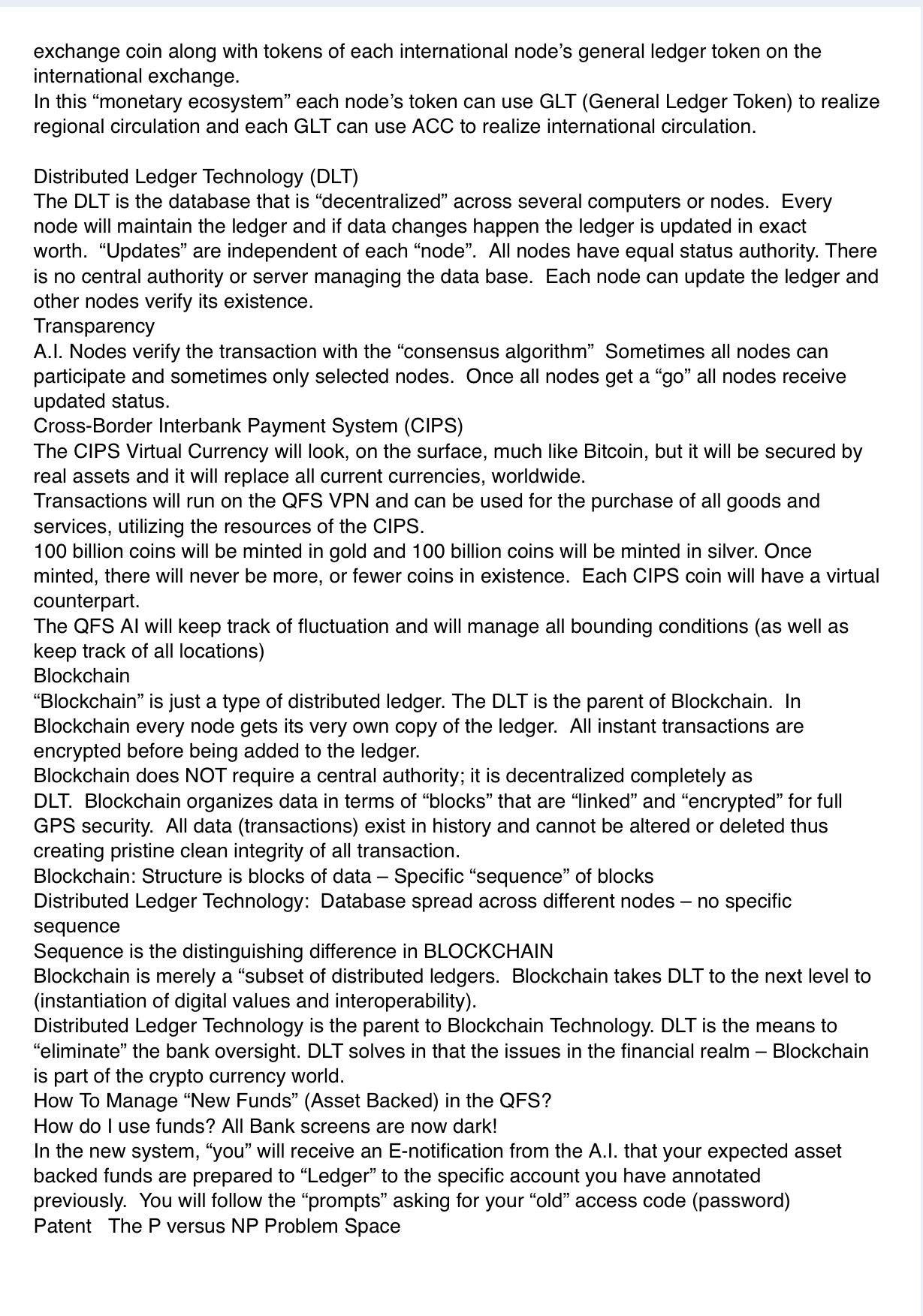The image captures an extensive and detailed webpage dedicated to explaining various financial and blockchain technologies. It provides comprehensive information about General Ledger Tokens (GLT) and Distributed Ledger Technology (DLT) while emphasizing DLT's foundational role in blockchain systems. The article also discusses the Cross-Border Interbank Payment System (CIPS) and elaborates on the Quantum Financial System (QFS) and QFS VPN. Additionally, it offers in-depth explanations on managing asset-backed new funds within the QFS and delves into the intricacies of blockchain technology and Non-Fungible Tokens (NFTs). The page is densely packed with detailed definitions, descriptions, and the significance of names and symbols within this technological and financial ecosystem.